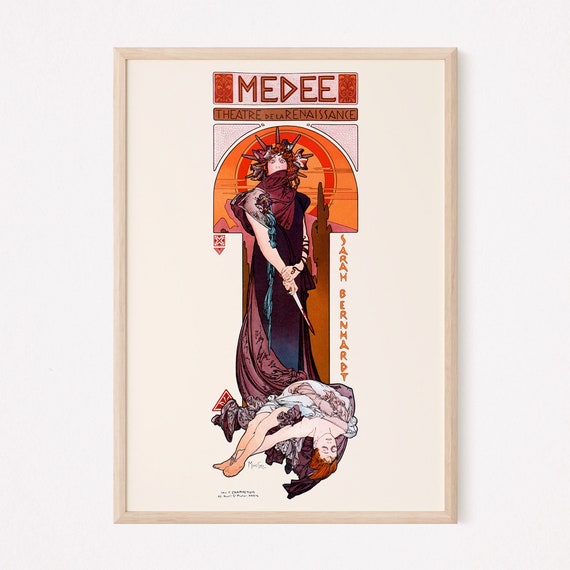This intriguing photograph captures a framed poster with distinct Art Deco elements. The poster announces "Medée" at the top, with the subtitle "Théâtre de la Renaissance" written in red lettering beneath it. The right side of the poster features the name "Sarah Bernhardt," possibly indicating the actress or character depicted. The central image showcases an intense and dramatic scene: a woman adorned with a sun-ray tiara and a red shawl, wielding a bloodied dagger. Behind her, an orange orb—reminiscent of the sun—casts a striking backdrop. At her feet lies another woman in a seemingly unnatural, lifeless posture, highlighting the violent encounter. Both women have striking red hair, enhancing the dramatic and mythological essence of the illustration, which evokes both Greek tragedy and elements of ancient civilizations.